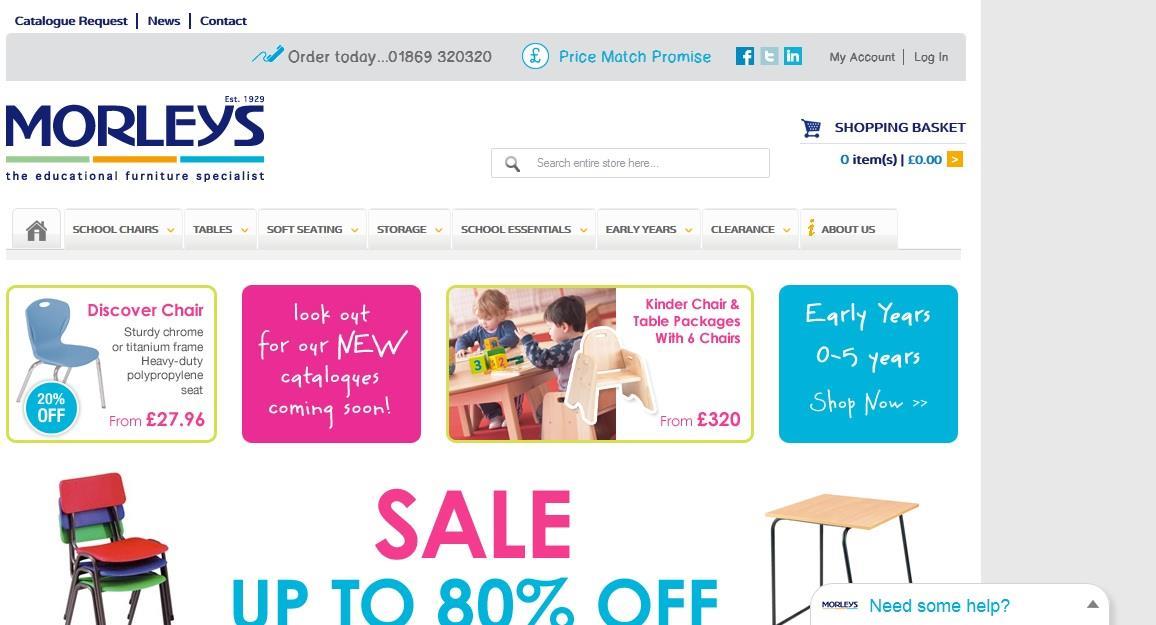**Educational Furniture Store Website - Morley's**

At the top of the website, a navigation bar features the following links in black text: "Catalogue Request," followed by a vertical line, then "News," another vertical line, and "Contact." Below this navigation, a horizontal grey strip spans the page, highlighted with a small blue telephone icon next to the text "Order Today: 01869 320 320". Adjacent to this are icons for Facebook, Tumblr, and LinkedIn, followed by "My Account" and "Login" separated by another line.

The header prominently displays the store name, "MORLEY'S," in dark blue, all-caps letters. Beneath the name are three horizontal lines in light green, dark yellow, and light blue. Under this, the tagline reads: "The Educational Furniture Specialist".

Several advertisements are arranged below the header. On the left, an ad for the "Discover Chair" priced at £27.96, offers a 20% discount and highlights features like a sturdy chrome or titanium frame and a heavy-duty polypropylene seat. Next to it, a pink block promotes "Look out for our new catalogues coming soon" in white text.

To the right of these ads, an image shows two young children with blonde and dark brown hair playing with blocks at a small wooden table. The caption reads, "Kinder Chair and Table Package with six chairs, £320". Nearby, a blue block indicates "Early Years, 0-5 Years, Shop Now".

At the bottom, a bold proclamation in bright pink states "SALE: Up to 80% off" in light blue, all-caps lettering. To the left, a picture shows three stacked chairs in red, blue, and green. On the far right, an image displays a school bench or desk with black iron legs and a faux wooden tabletop.